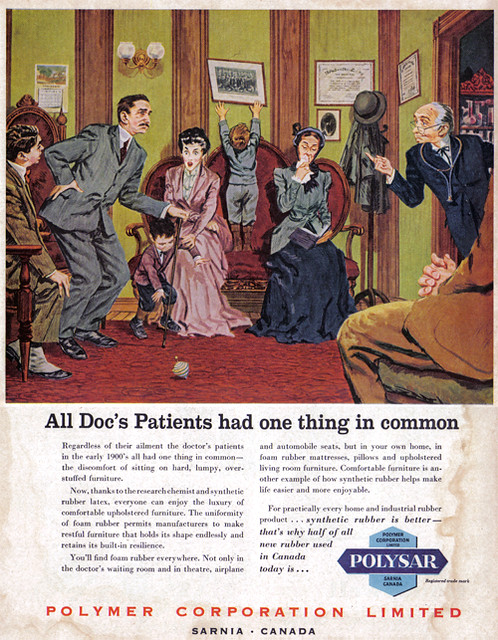In this vintage color advertisement, the central scene portrays a doctor's waiting room from the early 1900s, vividly brought to life with intricate details. The room features brown wooden columns set against a pea green wall with narrow vertical bands in between. A red sofa takes center stage, where a little child stands, mischievously reaching up toward a painting on the wall. Two women dressed in 19th-century attire flank the child; one in a pink dress has a young child at her feet playing with a top on the red carpeted floor, while the other coughs into a handkerchief. Nearby, a man stands awkwardly with a crooked back and bent knees, emphasizing the general discomfort shared by the doctor's patients. A doctor, adorned with a stethoscope around his neck, points towards one of the individuals. Beneath this scene, a headline reads, "All Doc's Patients Had One Thing in Common." Four paragraphs of black text follow, discussing the advancements in comfort brought by synthetic rubber latex, attributed to Polymer Corporation Limited. The bottom section prominently features the company’s name in red, "Polymer Corporation Limited," along with "Sarnia, Canada" in black, and a blue logo with the word "PolySAR." This ad highlights the improved comfort and durability of modern upholstered furniture, thanks to foam rubber innovations.